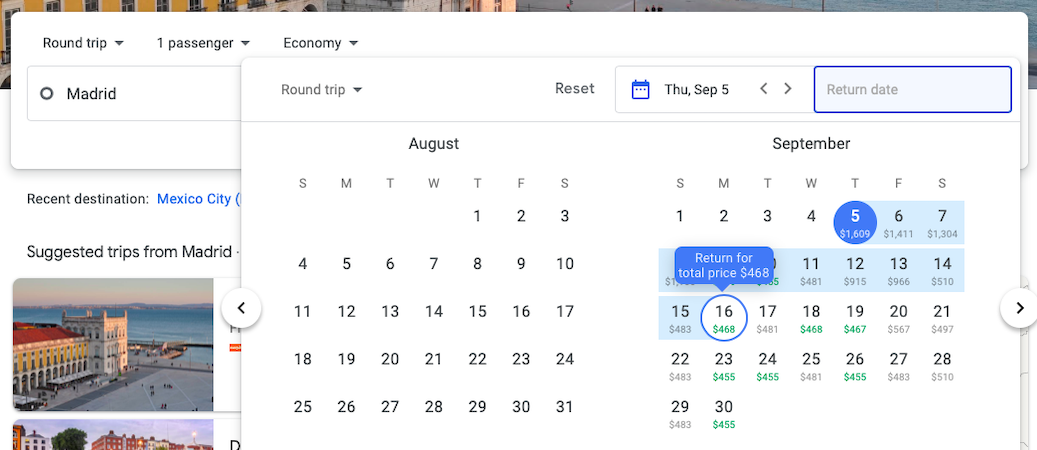This image captures a travel-themed web page showcasing various elements related to trip planning and booking. The primary screen of the web page displays eye-catching visuals, including two photographs of hotels located on serene beaches. One of these pictures vividly portrays a sunset scene, while the other image appears truncated and partially visible. Text on this main screen mentions “Suggested trips from Madrid” and highlights “Recent destination: Mexico City,” with the latter phrase appearing in clickable blue text.

In front of this main display, there are several overlapping pop-up windows adding layers of information. The initial pop-up at the top reads “Round trip, one passenger, economy,” and displays "Madrid" as the departure location. A larger pop-up window overlays this, presenting more detailed booking options: “Round trip” and “Reset.”

Significant detail is shown within this larger pop-up, where a user has input “Thursday, September 5th” as their departure date, but has not yet selected a return date. This date entry is highlighted in a blue box with gray text. Below the date entry, there are two calendars for the months of August and September. The August calendar appears with just the dates visible, while the September calendar shows a blue circle around the 5th. Dates from the 6th to the 15th are grayed out, and the 16th is outlined in blue.

Text at the bottom of the pop-up provides financial details: “Return for a total price of $468.” Additionally, near the September 5th date, there is another figure that seems to read either $1,000 or $1,609, though it is somewhat unclear.